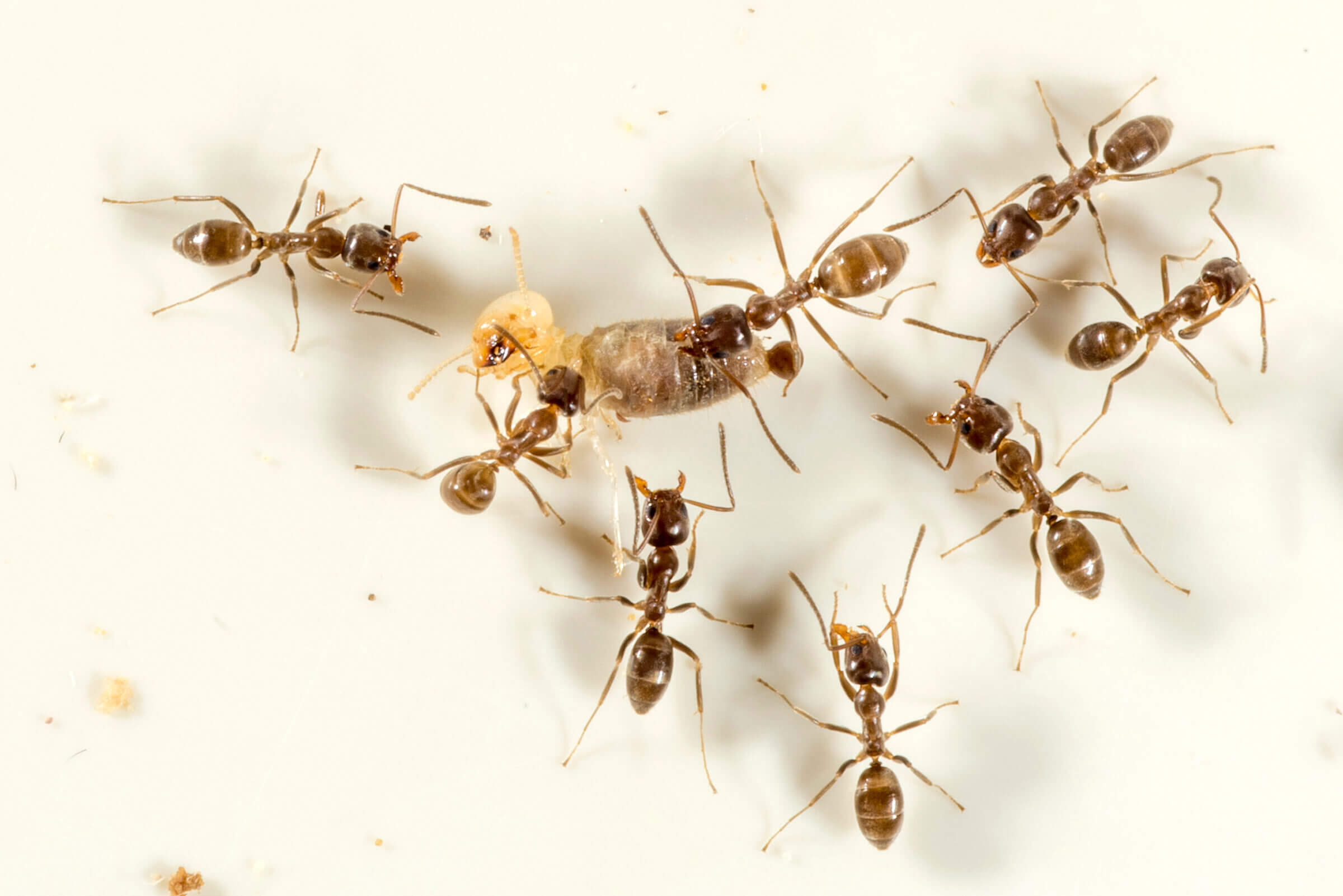In this close-up photograph, we see a white or off-white background dotted with small specks of food or dirt. Prominently displayed is a colony of eight brown ants with lighter brown stripes on their abdomens. Most strikingly, two ants are in the center, appearing to assist a larger translucent white insect, which might be a larva or the queen emerging from a cocoon-like structure. The ants are engaging in what seems to be a coordinated effort to handle or uncover this central insect, which is notably larger in width but similar in length to the ants. The composition includes approximately four ants on the right, one on the left, and one positioned below the central activity, showcasing a complex and intricate behavior within the ant colony.